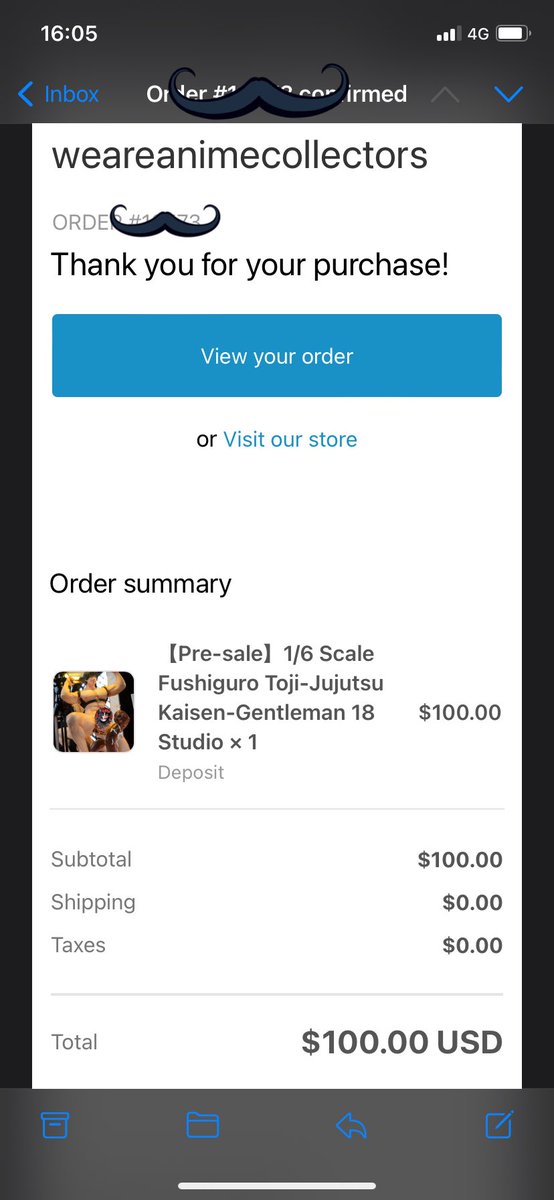Screenshot from an e-commerce website interface:

The top portion, approximately an inch wide, features a very dark gray, almost black, header. Thin black borders run down both the left and right sides, with a medium gray footer of about an inch across the bottom. The main background is white.

In the top left corner, the time is displayed as "16:05". To the right, the status icons show a full battery, 4G signal, and three out of four bars in white. Below the time, there is a blue greater-than sign pointing to the left, labeled "Inbox" in white lettering with a black mustache graphic curled at the ends covering part of the text. Visible letters include "O" on the left side of the mustache and "R M E D" on the right.

Further down, there is a greater-than sign pointing up in gray and one pointing down in blue. The main white section in the center displays text that runs together as a single string, "we are anime collectors," followed by "war order." Another word is partially obscured by a second black mustache graphic. Below this text, in bold black font, is "Thank you for your purchase!"

A blue rectangular button spans almost the width of the screen, with "view your order" in white text. Below this button, in blue, it says "visit our store." About midway down the page in black lettering is "Order Summary."

An image of an anime character appears below the order summary, with the character's name to the right and the price of "$100" further right. Directly beneath the anime character, a thin gray line delineates sections. To the left, it says "Subtotal," "Shipping," and "Taxes," while the respective amounts on the right are "$100," "0," and "0." Below these, it shows the "Total" on the left with "$100" on the right.

Within the gray footer section, there are several blue icons: a trash icon, a folder icon, a left-pointing arrow icon, and a square icon with a pencil. A white border stretches horizontally about an inch from the center to the left and right.